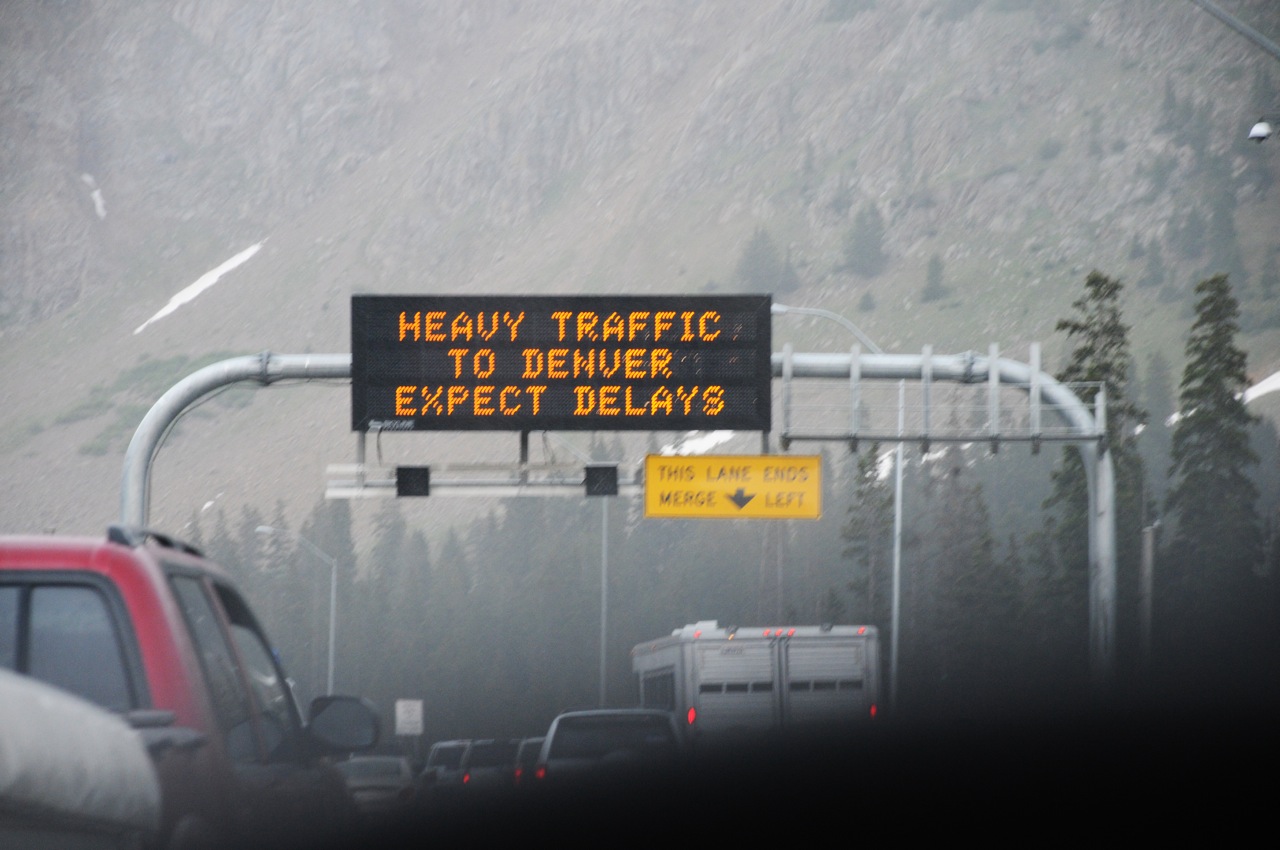The image depicts a multi-lane highway bustling with vehicles traveling in the same direction as the one from which the picture is taken. In the lower right corner, part of the image is obscured by a black object, likely the interior of the vehicle used to capture the photo. Prominently positioned just ahead and slightly to the left is a red pickup truck. To the right, there are approximately five vehicles, possibly including a mix of pickups and sedans. Farther to the right, there is a partially visible trailer or camper attached to the back of another pickup truck, though the limited view makes full identification difficult. 

Flanking the highway are stretches of evergreen trees, adding a scenic element to the busy road. Overhead, a sign mounted on a pipe supported by two vertical beams with rounded corners provides essential traffic information. The sign's letters are in bright orange on a black background. It appears to be a Dextronix brand sign, with a smaller, out-of-focus white-lettered section at the lower left corner. The main message reads, "Heavy traffic to Denver - expect delays." Just below this sign, two unlit lane control signals are visible. These signals are capable of displaying Xs to indicate closed lanes. To the right of these signals is another light orange sign with a black arrow pointing downwards, inscribed with the warning, "This lane ends - merge left."

In the distant background, the gentle slope of a mountain rises, giving depth and a sense of location to the image.